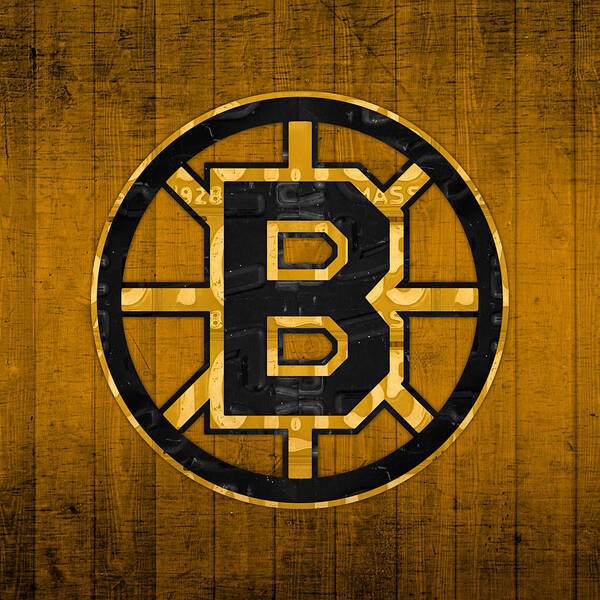This image showcases the Boston Bruins logo prominently displayed on a rustic, wood-paneled background. The wooden panels are tall, skinny, rectangular planks with a gradient effect, transitioning from a bright yellow or golden center to darker tones at the top and bottom edges, where a light film or mist of black is visible. This background gives a scratched and weathered appearance, enhancing the overall rustic feel. In the center, there is a distinctive circular logo. The outer ring of the circle is a thin yellow border, inside of which lies a thicker black border marred with touches of gray and white, giving it a textured look. Within this black ring is a large letter 'B,' rendered in black and bordered with yellow. From this 'B,' lines extend outward, connecting it to the circular border. Various numbers and letters, including "1928" and possibly "Massachusetts," appear in a translucent white font overlaying the logo, adding to the intricate design. The image appears to be computer-generated rather than a photograph, presenting a detailed and polished representation of the Boston Bruins emblem against the rustic wooden background.